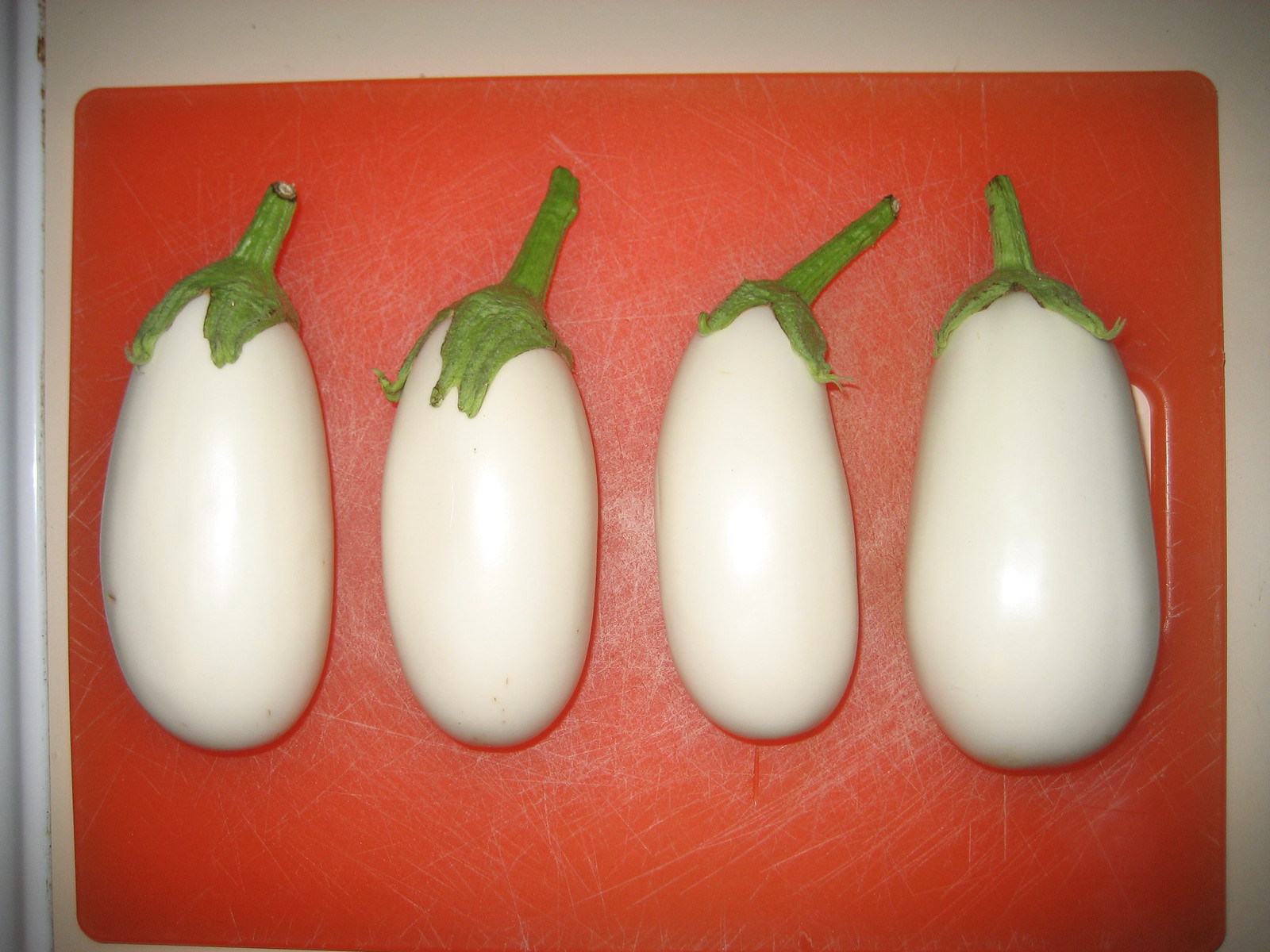In this photograph taken from a top-down perspective, the focal point is a bright orange plastic cutting board, heavily marked with cut lines, featuring a handle in the form of a hole on the right-hand side. Resting on this cutting board are four uncommon white eggplants, characterized by their ovular, oblong bodies, green stems, and tops. The cutting board itself stands out against a white tabletop, framed by a lighter gray border around the top, left, and right sides. The clean lines and distinct color contrasts create a visually striking image with meticulous attention to detail.